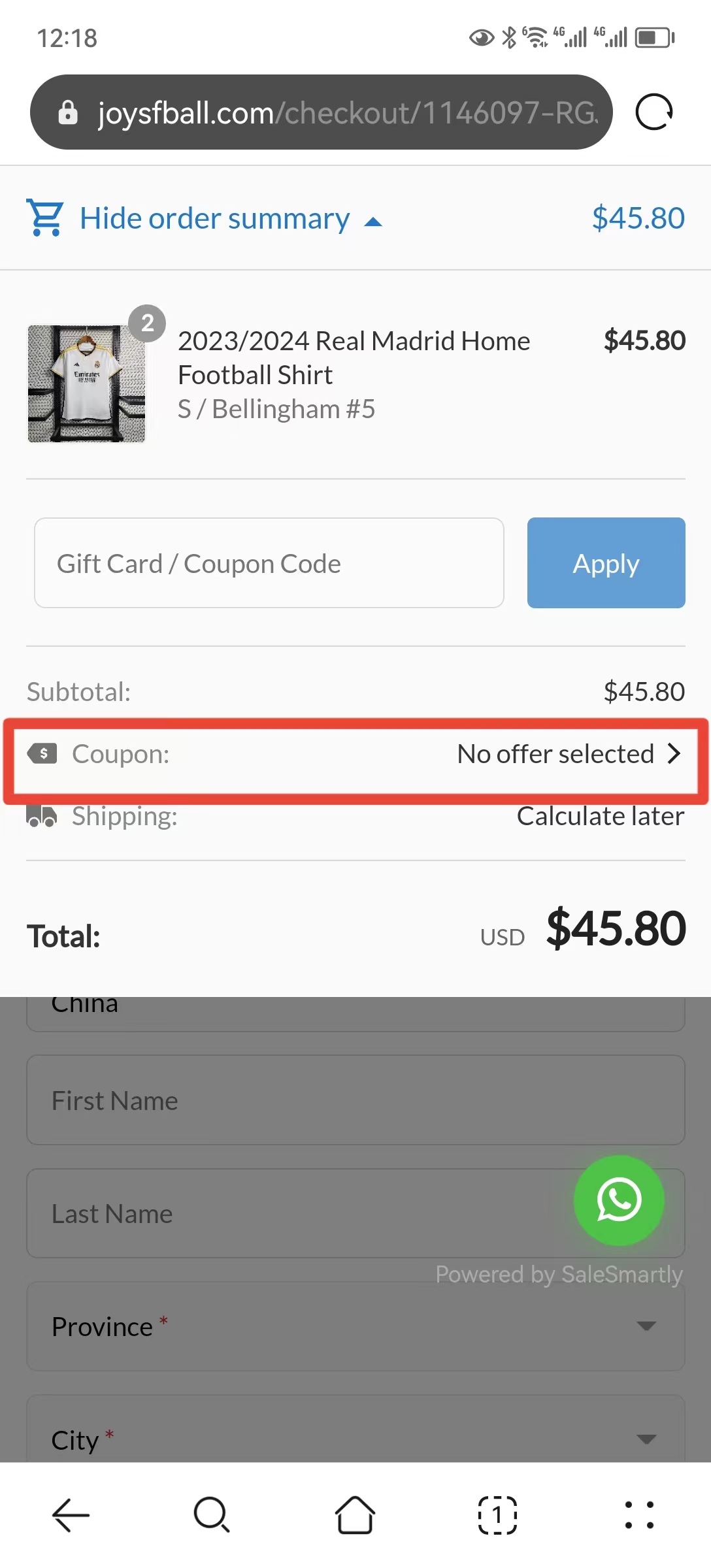Screenshot of a website viewed on a smartphone:

### Header Section:
- **Time and Status Icons**: 
  - *Left*: "12:18" in black on a white background.
  - *Right*: A series of black icons including:
    - An eye symbol.
    - Bluetooth icon.
    - Cell phone signal strength bars.
    - "4G" text alongside signal strength bars.
    - Battery icon.

### URL and Navigation:
- **Search Bar**: 
  - Black bar with a white padlock icon on the left.
  - URL "joysfball.com/checkout/1146097-RG" in white text.
  - Black semicircle refresh icon on the right.

### Main Content:
#### Order Details:
- **Order Summary Bar**:
  - Blue with a blue card icon on the left.
  - Text: "Hide order summary"
  - Price: "$45.80" in blue on the right.

- **Product Image and Details**:
  - *Left*: Image of a white shirt hanging on a tote hanger.
  - *Upper Right of Image*: Gray circle with white tube icon.
  - *Right of Image*: 
    - "2023/2024 Real Madrid Home football shirt S/Bellingham number 5" in black text.
    - Price: "$45.80" in black text.

- **Payment and Coupons**:
  - *Below Product Details*: 
    - Search bar labeled "Gift card/coupon code" with a blue "Apply" button.
  - *Subtotal Section*:
    - "Subtotal" in black text with corresponding price "$45.80" also in black.
  - *Coupon Section*:
    - "Coupon" in black text.
    - "No offer selected" in black, all surrounded by a long red bar.
  - *Shipping Section*:
    - "Shipping" in black text with "Calculate later" to the right.
  - *Total Section*:
    - "Total" in black text with "USD" in gray.
    - Final price: "$45.80" in black text.